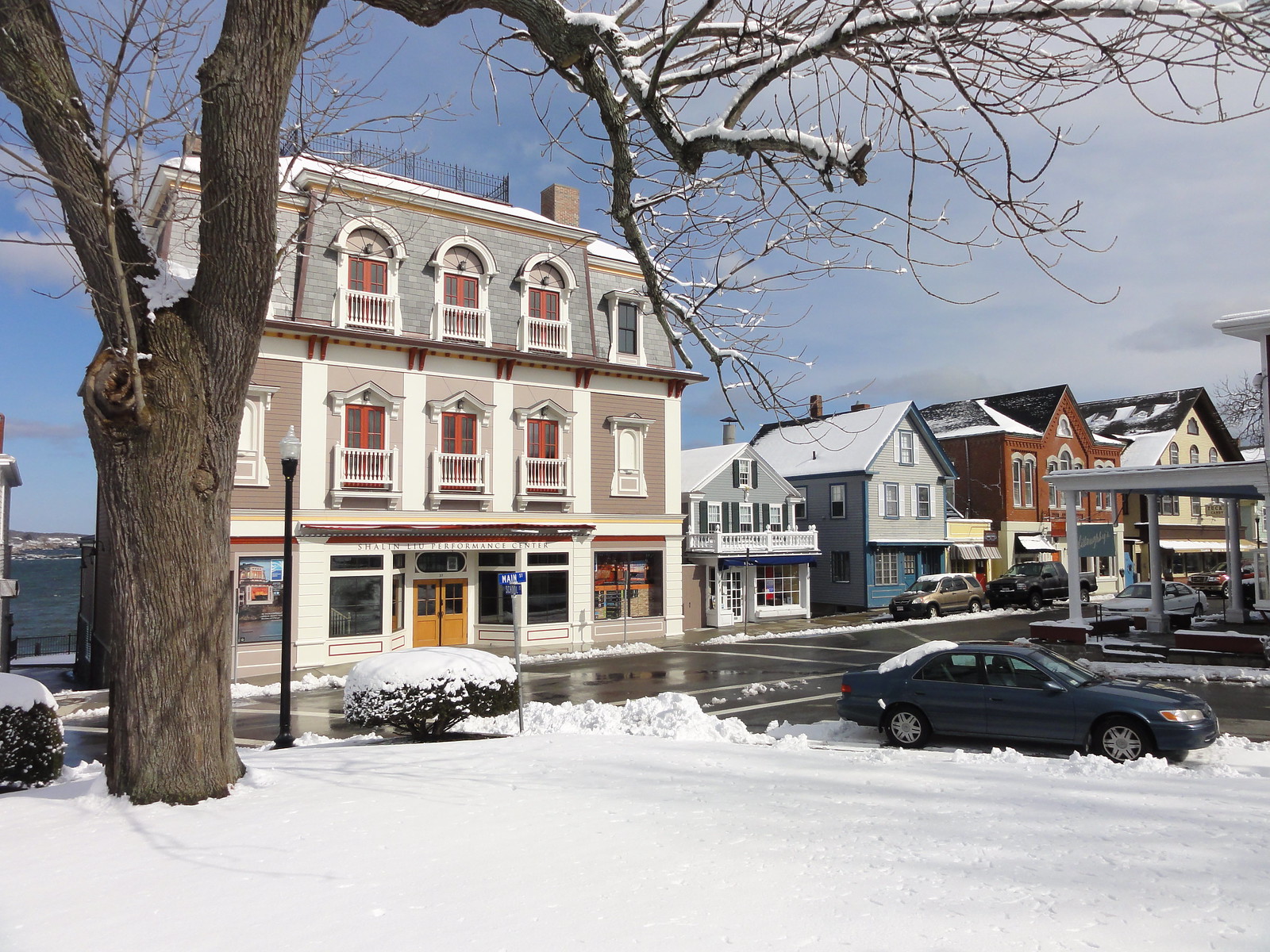In the well-preserved town, reminiscent of early 1900s New England architecture, stands a meticulously maintained three-story building. Central to the upper two floors, accessible through exterior doors, is a flat, mid-century style balcony. Bold lettering announces the "Shalin Liu Performance Center" on the front façade. Adjacent to this cultural hub, a series of equally well-kept buildings line the street, exuding a clean and inviting charm.

The foreground is blanketed in a pristine layer of snow, contrasting beautifully with the cleared street in the middle of the photograph. This plowed area reveals part of an intersection where a single car is parked, suggesting recent activity. Additional vehicles can be seen parked along the right half of the image, adding to the scene's bustling yet serene atmosphere.